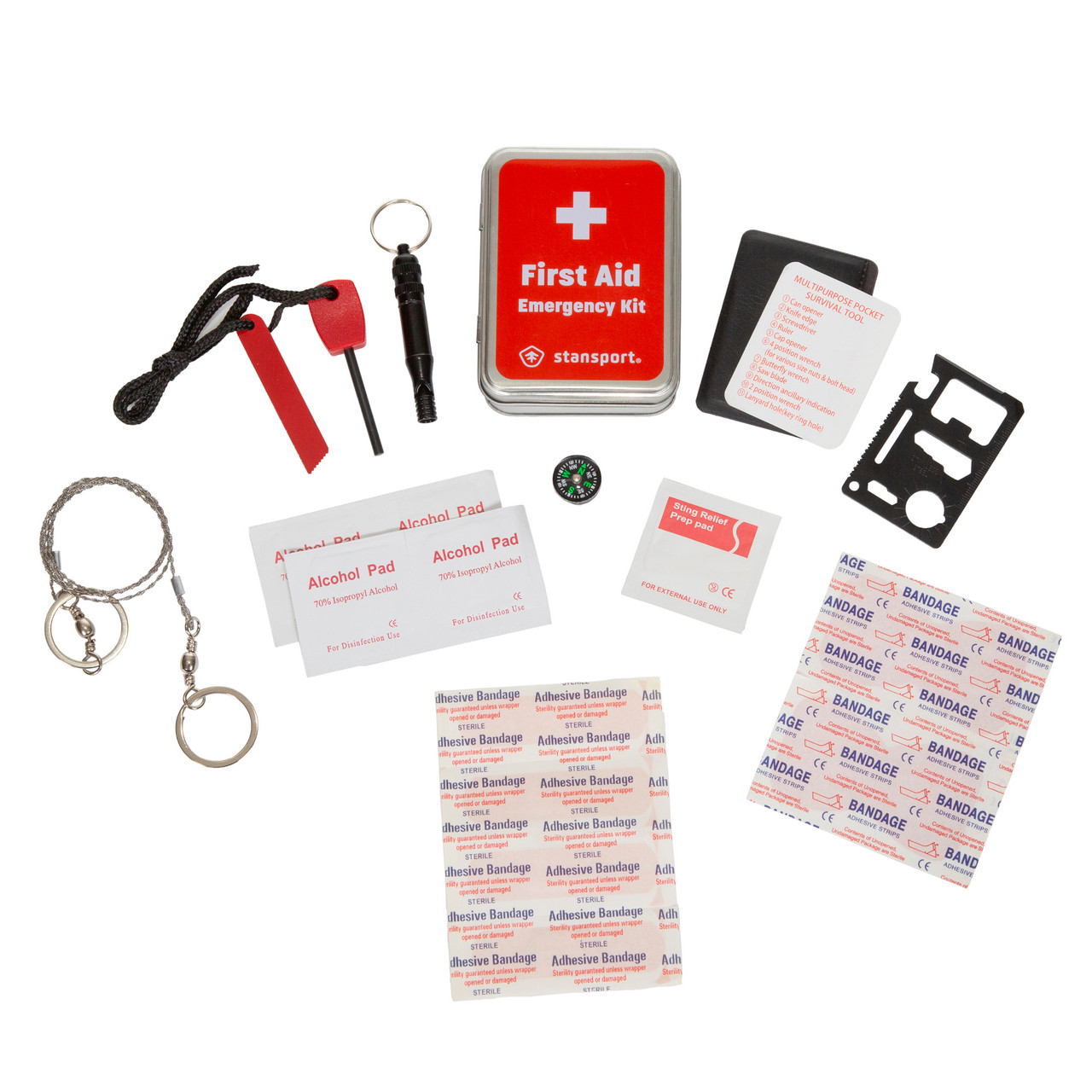This image is a flat lay display typical of an Amazon product listing, showcasing a first aid emergency kit with all its components neatly spread out on a completely white background. The centerpiece at the top is a rectangular metal box, silver in color with a red lid featuring a white cross and the words "first aid emergency kit", along with the brand name "Stansport" at the bottom. Spread around the main kit are several notable items: adhesive bandages in white packages with blue and red text, a set of four white, rectangular alcohol pads, and various other first aid tools. Among the spread, there are also a few black and red tools, a keychain with rings attached, and a mysterious circular green item along with a black object that appears to have sections cut out of it. The meticulous arrangement and clear presentation make it easy to see the contents and understand what you'd receive when purchasing this first aid kit.